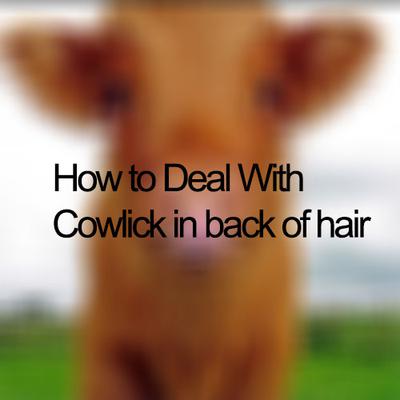The image features an out-of-focus brownish-red cow positioned in the center, facing the camera with its pink nose and dark eyes faintly visible. The cow's ears stick out to either side of its head. The backdrop is indistinct but suggests a green grassy field below a blue sky occupying the top three-fourths of the frame. Superimposed on this blurred pastoral scene is black text reading, "HOW TO DEAL WITH COW LICK IN BACK OF HAIR." The text is prominent and in the middle of the image, with the words "how," "deal," "with," and "cow lick" capitalized. The purpose of the image appears to provide instructions on managing a cowlick hairstyle, using the cow as a visual pun.